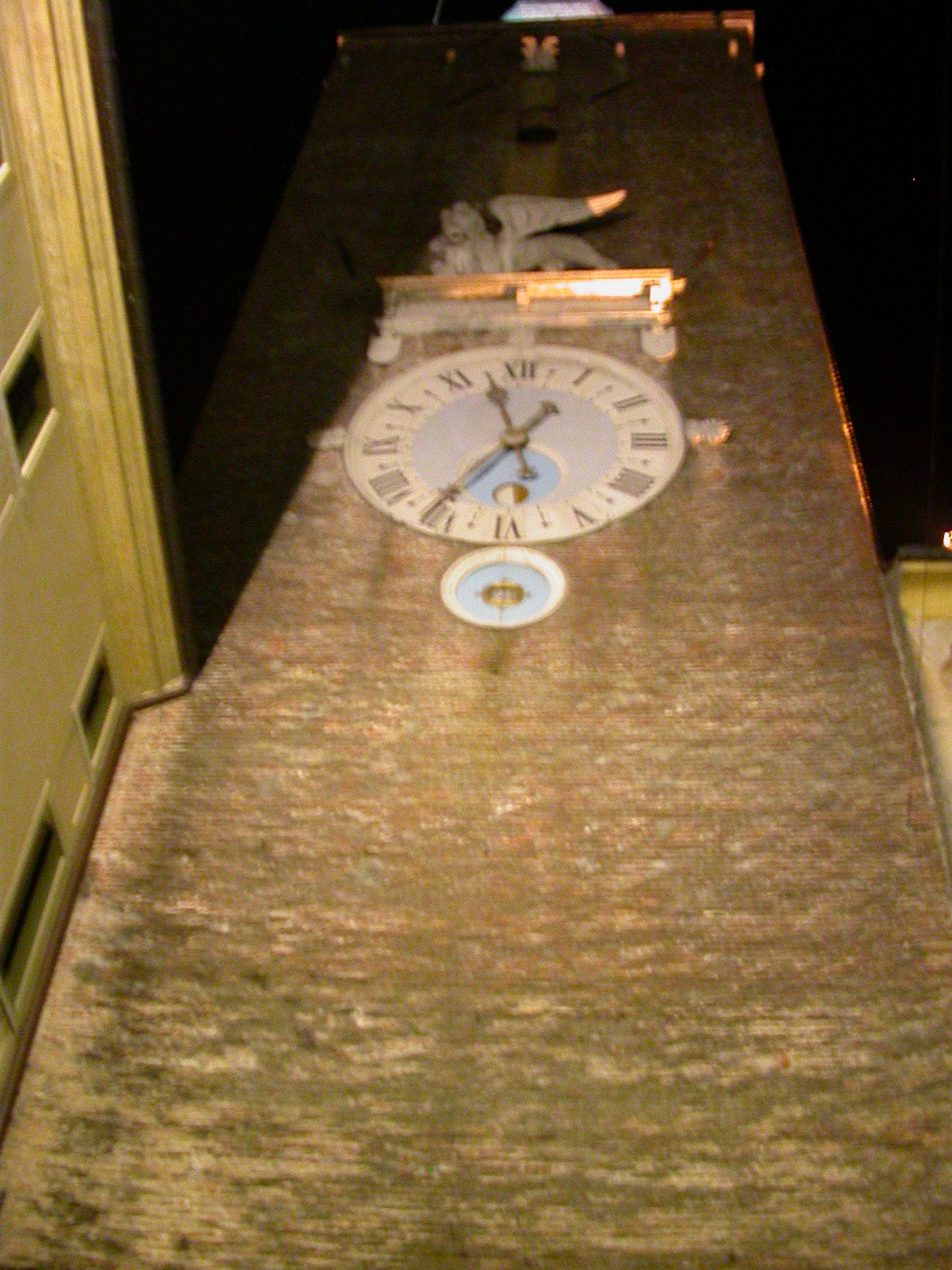This vertically rectangular, exterior nighttime image appears blurry and pixelated, likely due to its capture in low light conditions. The main focus is a very tall stone tower, with a surface that shows a mix of brownish and greenish hues. Prominently featured on the tower is a large, antique-looking clock with a white face, Roman numerals, and brass-colored hands, indicating approximately 20 minutes to midnight. The clock is set into the side of the tower, which is flanked by buildings that cast partial shadows upon it. Above the clock, perched on a stone ledge, is a gray gargoyle-like statue with a wing extending from its back. The surrounding sky is pitch black, emphasizing the nocturnal setting and the dim lighting slightly illuminating the clock and parts of the tower.